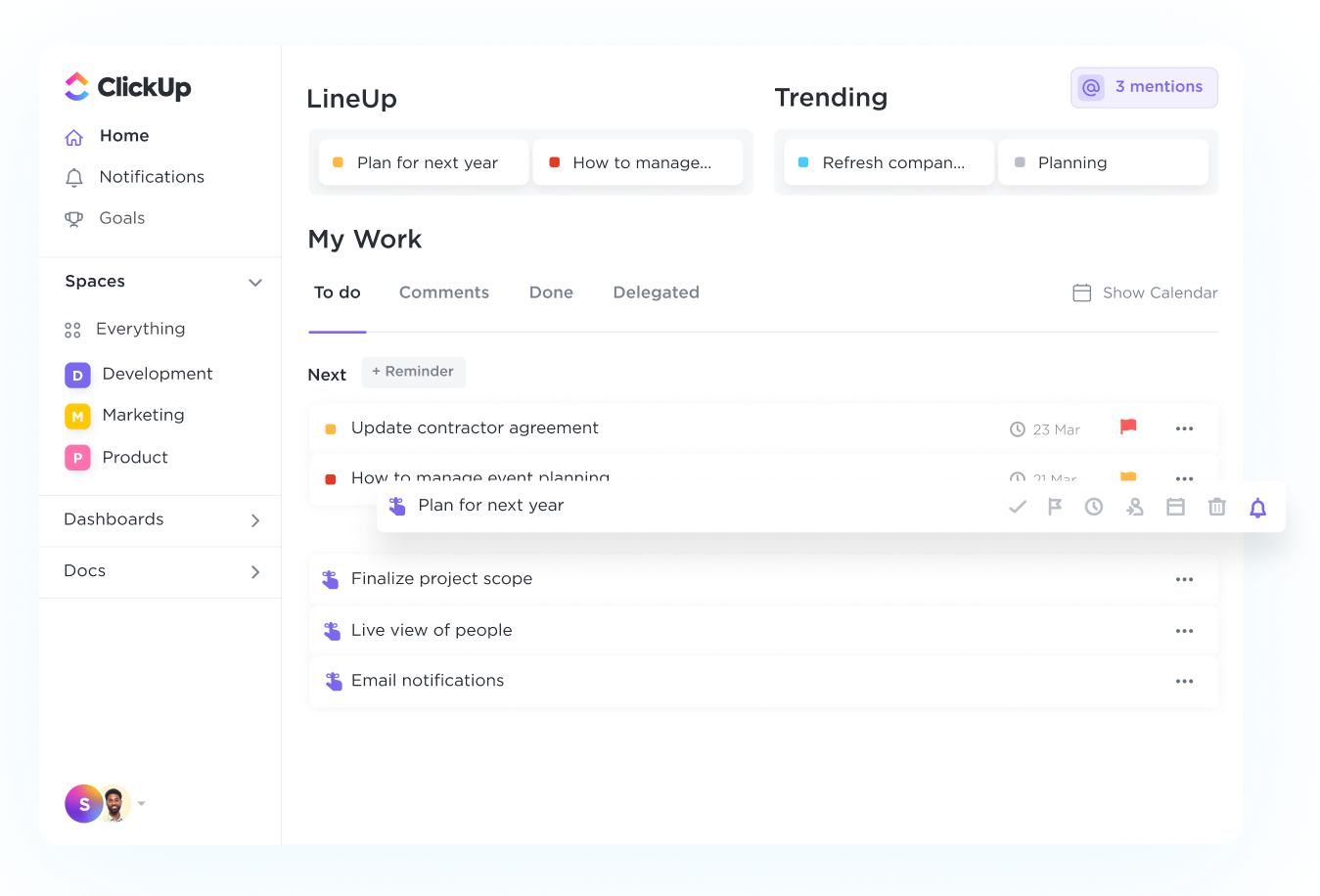This is a detailed screenshot of the ClickUp interface. In the top left corner, the "ClickUp" logo is prominently displayed in black font, accompanied by a distinctive logo featuring a red upward arrow and a blue semicircle positioned below it, both elements not touching. A vertical menu is situated on the left side of the interface, directly below the logo. This menu includes the sections: Home, Notifications, and Goals. Following these, the menu lists several Spaces, specifically: Everything, Development, Marketing, and Products. Further down the menu, options for Dashboard and Docs are visible.

Moving towards the central area of the interface, the top section is labeled "Line Up." Directly below this heading, there is an entry titled "Plan for Next Year," followed by another labeled "How to Manage." To the right of these entries, there is a section marked "Trending." Underneath "Trending," there is a button labeled "Refresh Company," followed by another segment titled "Planning."

In the lower portion of the interface, there is a section called "My Work," which features multiple tabs. The "To Do" tab is currently selected, indicating the tasks to be addressed. This meticulous organization of sections and tabs within ClickUp provides a comprehensive overview of various projects, tasks, and planning tools available to users.